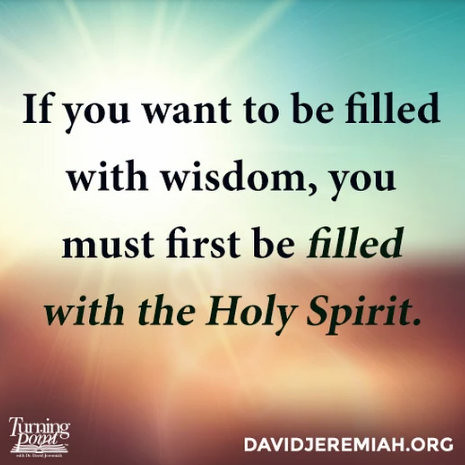The inspirational poster features a serene sunset with a gradient background transitioning from a light turquoise blue sky at the top to shadowy brown earth tones at the bottom. At the center of the image, a radiant white light bursts outward, adding a heavenly glow. Bold black text in a sans-serif font conveys the motivational quote: "If you want to be filled with wisdom, you must first be filled with the Holy Spirit." Emphasizing certain words, "filled" and "with the Holy Spirit" are in italics. In the bottom left corner, the logo for "Turning Point" is shown as an open book with its pages turning. The bottom right corner features the website davidjeremiah.org in all capital white letters.